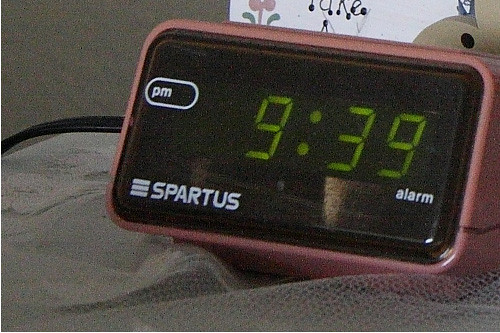The image depicts a close-up of a rectangular, old-school style digital alarm clock, predominantly colored in pink plastic with an indented line around its edge that creates a darker shade of pink. The face of the clock is black, prominently displaying the time as 9:39 in green digital numbers. On the left side of the clock face, an oval outline in white contains the letters "PM." Below the time display, "SPARTUS" is written in capital letters above the word "ALARM" in smaller letters. A black cord extends from the left side of the clock, indicating it's plugged in. The clock rests on a light gray surface, with a background that includes glimpses of a white and pink area and a portion of a brown wall.